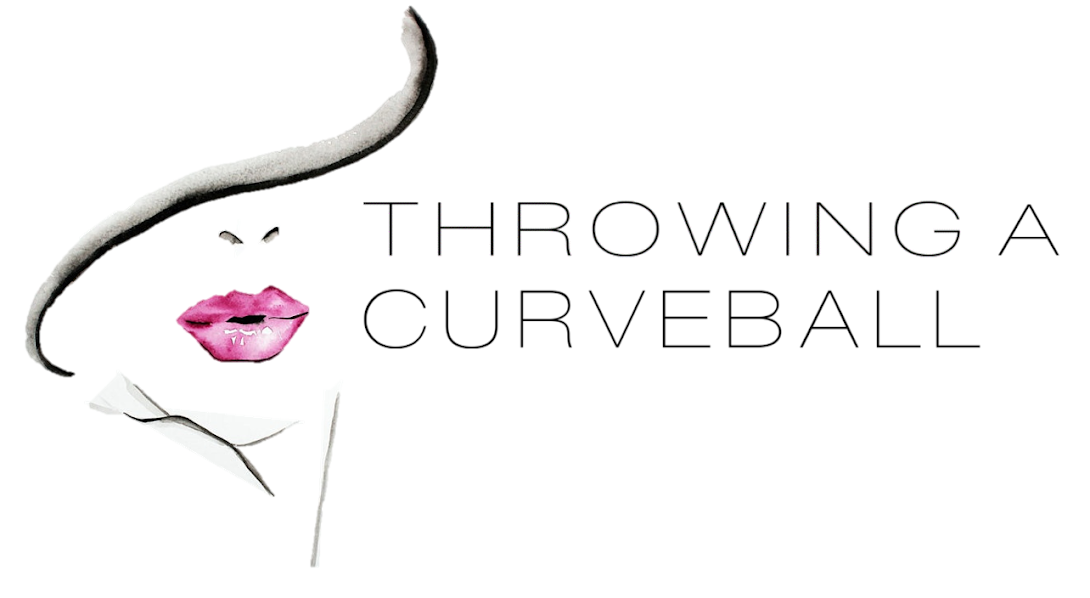The image appears to be a minimalist advertisement set against an all-white background. The primary focus is on two lines of text positioned on the right two-thirds of the image, written in all capital letters with thin black text. The top line reads "THROWING A" and directly below it is the word "CURVEBALL." These lines are left-justified.

To the left of the text is an artistic illustration of a woman's face, specifically the lower half, rendered in simple black and gray lines. The woman's eyes are obscured by a curved hat or shadow, revealing only her black oval-shaped nostrils. Below her nostrils, there are strikingly bright pink, slightly parted lips, which stand out as the only colorful element in the composition. The illustration continues with gray lines suggesting the contours of her chin and shoulders, enhancing the minimalist yet striking design of the ad.